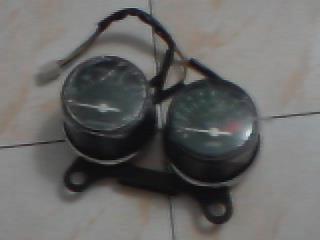The photograph features two cylindrical gauges centrally positioned on a flat, tiled surface. The image is rectangular, with its longer sides running horizontally. The tiles are a checkerboard pattern of white and peach hues, separated by thin black grout lines that converge underneath the gauges, creating an intriguing focal point. 

The gauges are mounted on a triangular-shaped metal bracket, which has two mounting holes at its base. Each gauge boasts a sleek, black, and metallic frame, secured onto a circular, silver-colored base. Semi-dirty transparent coverings protect the face of the gauges, allowing visibility of the intricate details beneath.

The gauge faces feature white numbers, notches, and needles, all designed for precision. Both needles are angled towards the bottom left, suggesting a possible reading or calibration state. Emerging from the top of each gauge are wires encased in black insulating material, terminating in a white plug, adding a sense of utility and connectivity to the overall visual narrative.